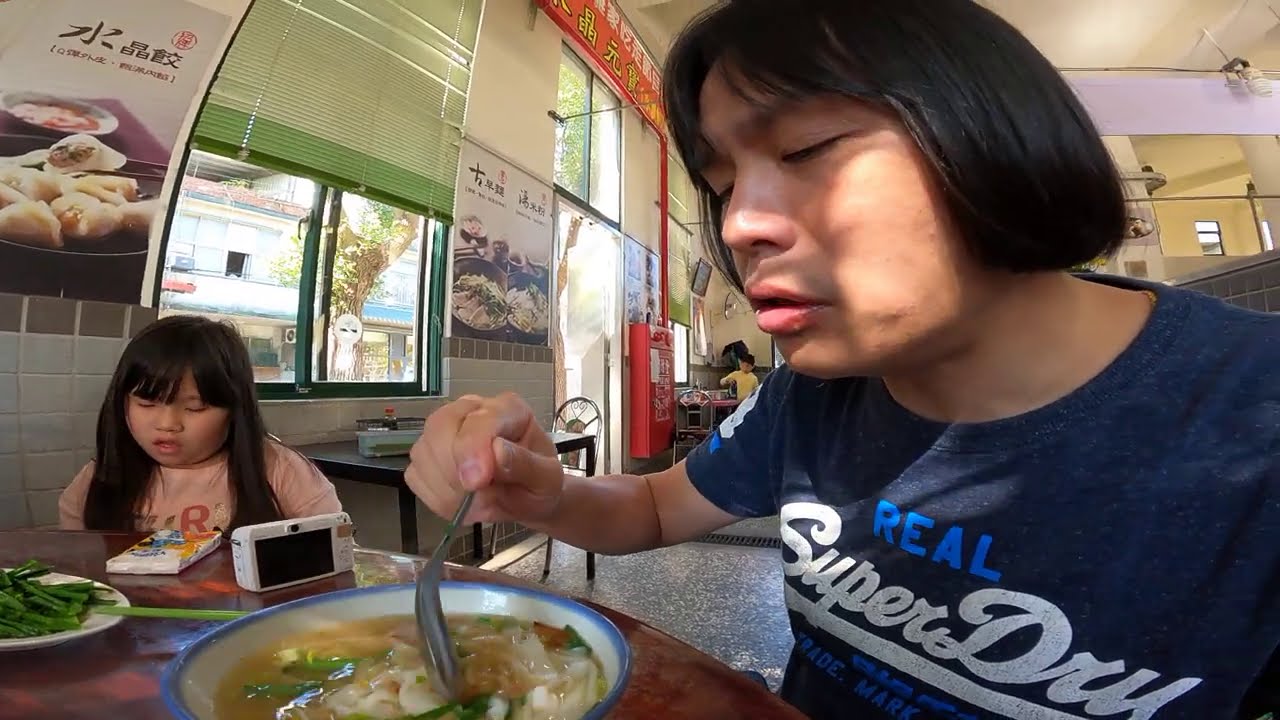This image captures an Asian family at a restaurant, with a young man and a girl prominently featured. The young man, sporting a mushroom-like haircut and wearing a blue t-shirt that reads "real super dry," is eating soup with a rather large metal spoon from a white porcelain bowl with a blue rim. The girl, who looks about 12 years old, sits beside him, focused on a book in front of her. There's also a plate of string beans on the table, and beside it, a white digital camera. The background features a poster with food advertisements and Chinese writing, showcasing dumplings with red sauce. The restaurant, characterized by white stone brick walls and high ceilings, appears busy, with another child visible at a distant table. Outside the windows, more businesses can be seen, contributing to the bustling atmosphere.